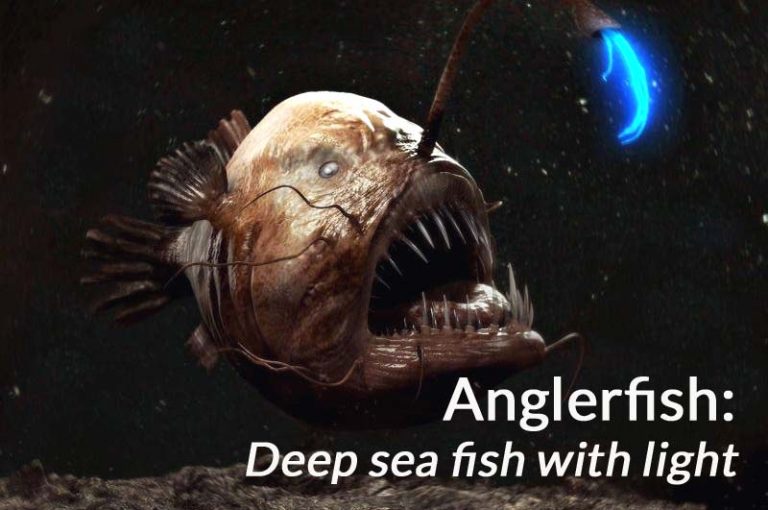In the deep, dark depths of the ocean, a terrifying angler fish dominates the center of the image. The background is a pitch-black void speckled with what looks like white dust particles, adding to the eerie atmosphere. The angler fish, with its mostly tan and brown coloration, seems almost prehistoric. Its disproportionately large head features long, razor-sharp teeth, and its eyes are eerily white. A distinctive appendage extends from the front of its head, resembling a tentacle or branch, at the end of which glows a blue light—its built-in lure for attracting prey. The fish's skin appears smooth, lacking the visible scales typical of other fish, and its body is equipped with a few fins and smaller tentacles. Below the fish, the ocean floor is partially visible, appearing either sandy or rocky, with some floating particles adding to the scene's depth. Overlaying the bottom left of the image is white text reading "angler fish: deep-sea fish with light," underscoring the unique and menacing features of this deep-sea dweller.